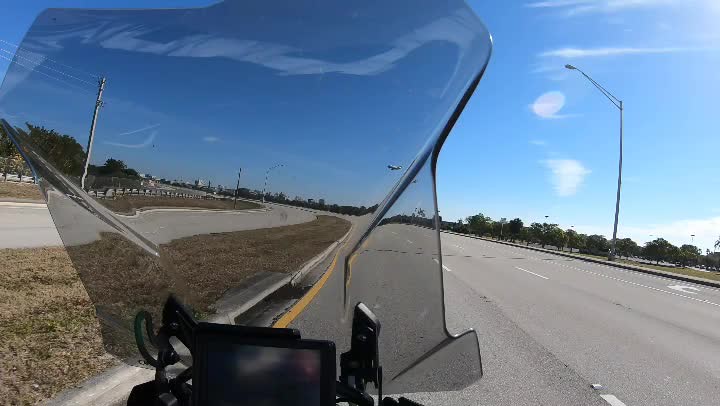The image depicts a point-of-view shot from a stationary motorcycle positioned on a highway. The motorcycle features a large, smoky-colored windscreen that shades the view from the sun. The highway consists of multiple lanes, with at least three lanes in the direction the motorcycle is facing, including a turn lane on the far right. Separating the lanes for opposing traffic is a grassy median strip. The scene is illuminated by a bright sun situated in the top right corner of the image, casting glares and highlighting a largely clear blue sky with some small streaks of white clouds. Bordering the highway are rows of trees and street lamps, which are not in use. The overall setting suggests a sunny day with minimal clouds, enhancing the visibility of the green median and surrounding landscape.